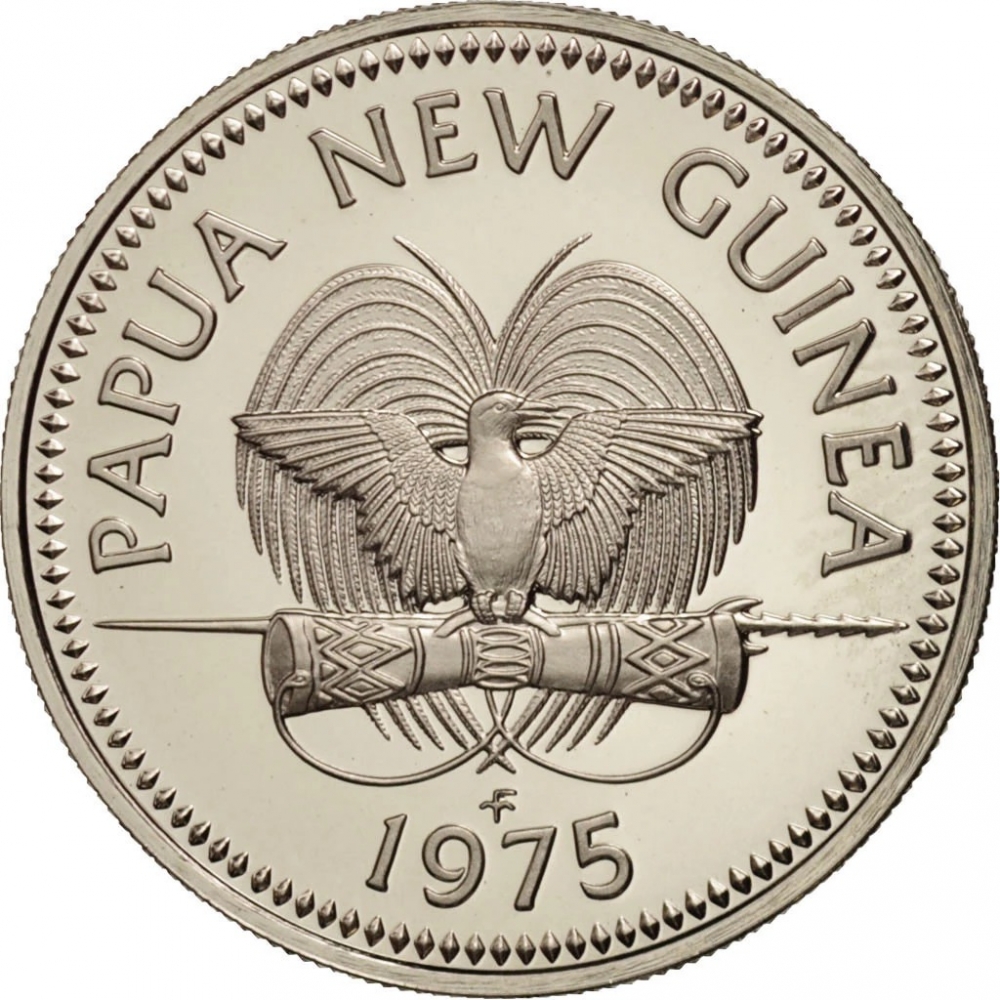This close-up image showcases the reverse side of a round, silver-gray coin from Papua New Guinea dating back to 1975. The coin features an intricate border decorated with raised diamond-like shapes which would be tactile if touched. At the top center, the words "Papua New Guinea" are elegantly curved. Dominating the central field of the coin is an exotic bird with an elongated bill and widespread wings, perched atop what appears to be a set of traditional wrist guards or a rolled-up scroll held by its feet. Fronds from a plant extend behind the bird, adding to the detailed design. Below this central figure, the year "1975" is clearly inscribed, with a small letter "F" above it, completing the intricate and symbolic imagery of this beautiful collectible.